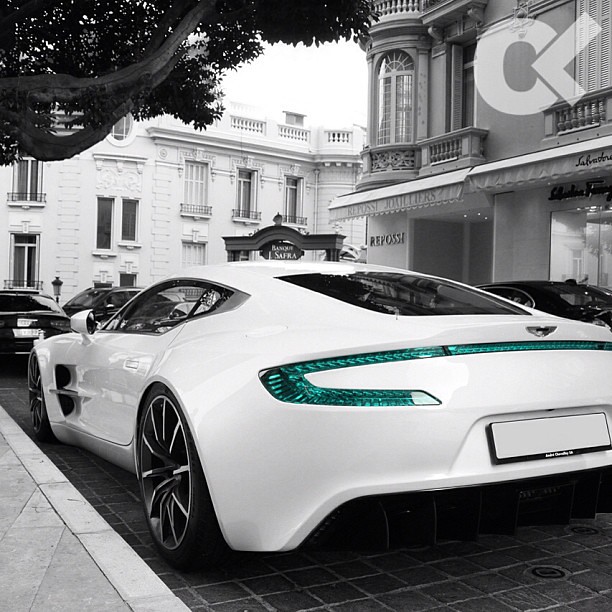The black and white photograph captures an outdoor urban scene dominated by an expensive-looking, modern white sports car positioned prominently in the center. The car’s distinct features include a striking strip of greenish-teal lights at the back, adding a pop of color to the monochrome setting. The license plate is obscured by a white block, rendering it unreadable. The vehicle is parked atop a roadway that appears to be paved with black tiles, bordered by a white curb and a nearby sidewalk in the lower left-hand corner. Surrounding the white car are several other vehicles, notably a black car to its right and another black car directly in front of it. A large multi-story white building with numerous windows looms in the upper part of the image, while the upper right-hand corner reveals a grayish building featuring half-moon windows and balconies. The upper left-hand corner is framed by overhanging tree branches and leaves. Notably, a building to the left displays a sign reading "Raposi" and resembles a luxury hotel. Additionally, a small white watermark featuring an O with an L inside is visible in the top left-hand corner.